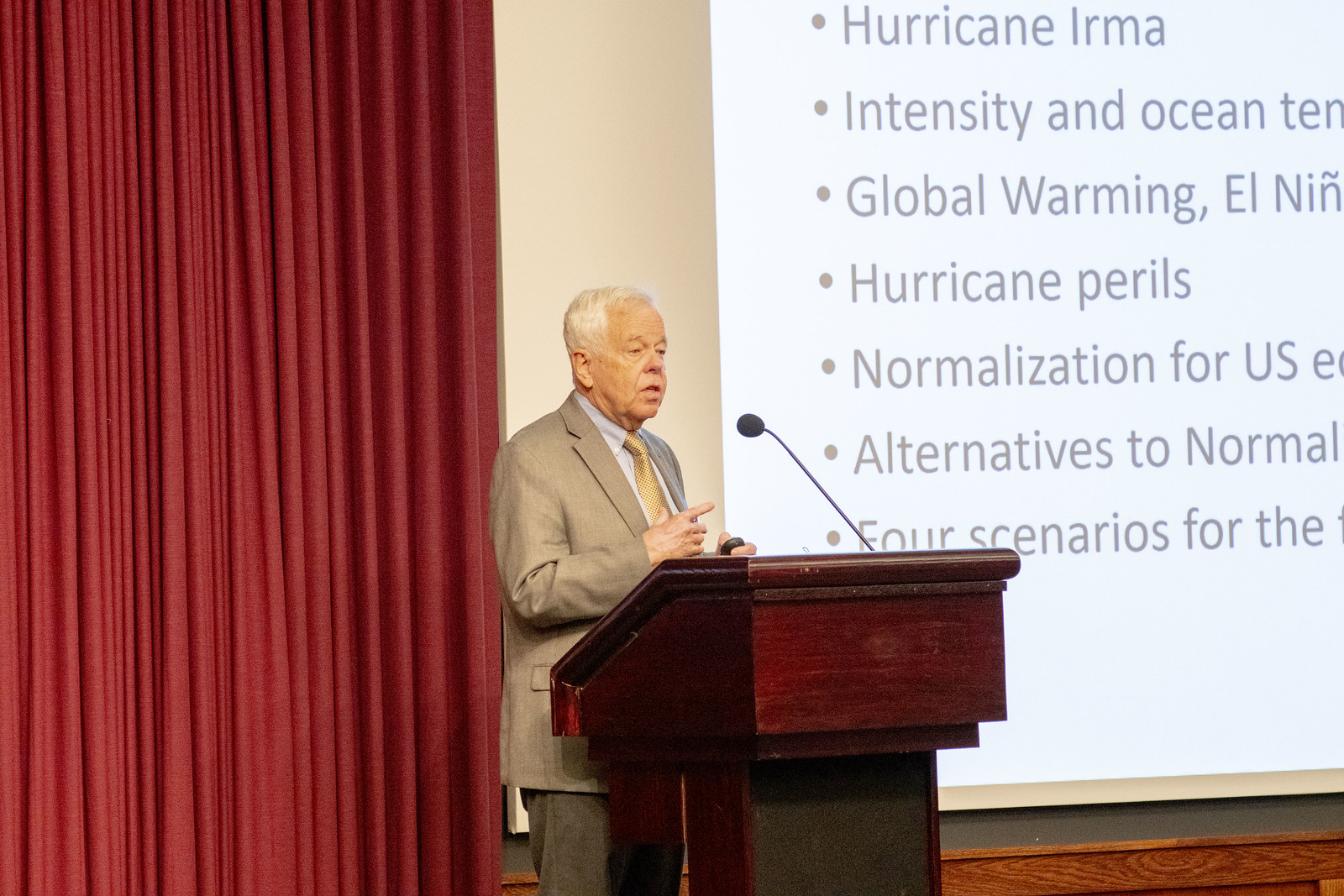In this image, an older man, possibly in his 60s or 70s, is delivering a lecture on stage. He stands behind an old, reddish-brown wooden podium, equipped with a microphone pointed towards his mouth. His attire includes a light tan suit coat, a light blue button-up collared shirt, a beige tie, and deep gray pants. The gentleman has short white hair, with some balding, and wrinkled skin.

Behind him, there is a long red curtain that is pushed back, likely used to cover the screen when not in use. To his right, a large white projector screen displays a PowerPoint slide with mostly black text, although the complete text isn't fully visible. The legible parts of the slide include phrases such as "Hurricane Irma," "Global Warming," "El Nino," "Hurricane Perils," "Normalization for U.S.," "Alternatives to Normal," and "forced scenario." These phrases suggest that the lecture focuses on topics related to global warming and climate change. The stage is set to convey a serious, academic atmosphere as the older gentleman engages with his audience.